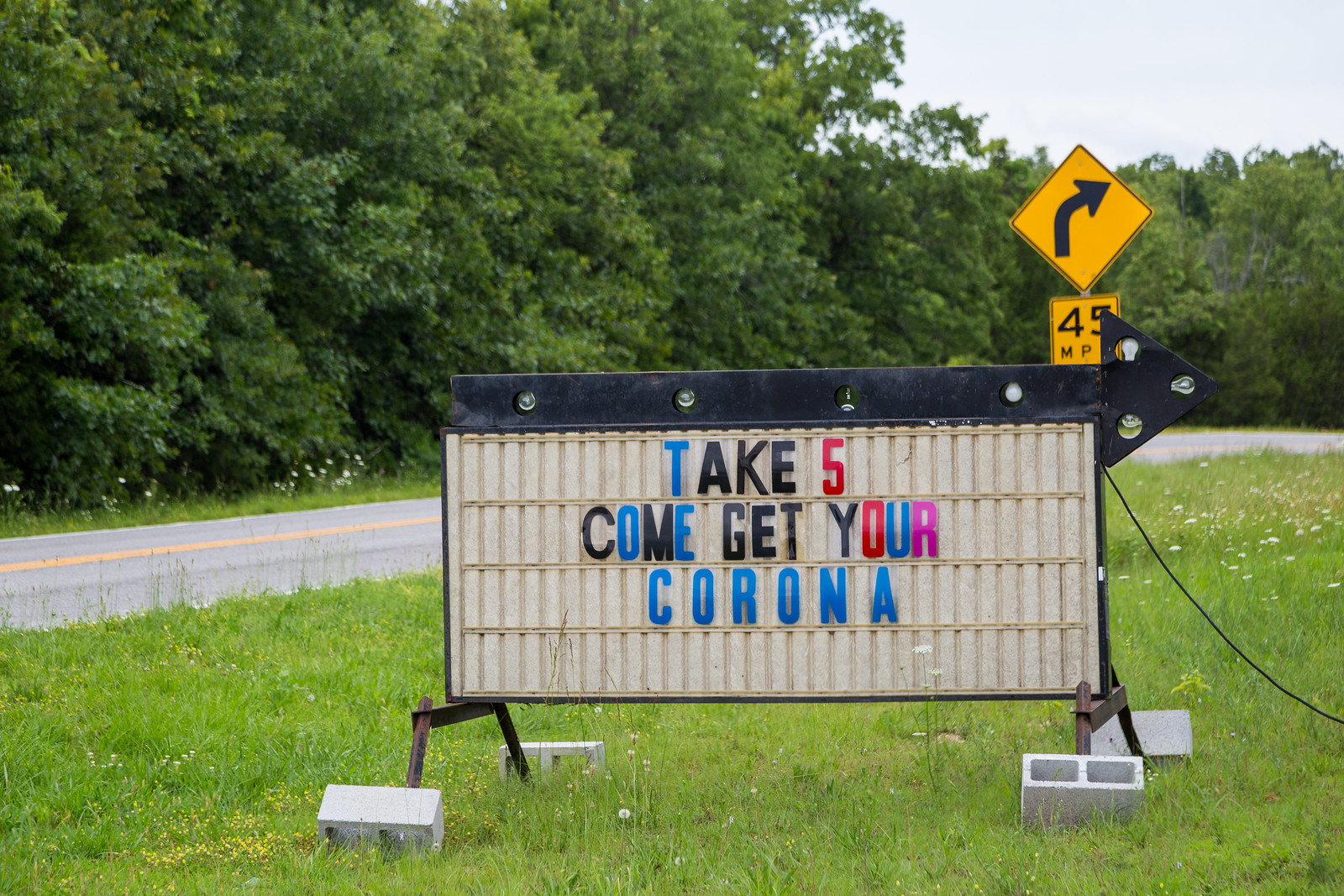In the foreground of this image, there is a black changeable copy sign featuring a black metal arrow with light bulbs, pointing to the right. The sign's main frame has an off-white background with yellow dividers, displaying the message in blue, black, red, and pink letters: "Take five. Come get your Corona." The sign is stabilized by four dark brown metal legs, each of which has a grey cinder block leaning against it. Surrounding the sign is an overgrown grassy area. Just behind this sign, there is a yellow diamond-shaped traffic sign indicating a right turn with a speed limit of 45 MPH in black letters. Further back, a grey road with a yellow line running down the middle stretches across the scene, and in the further distance, a lush green forest serves as a natural backdrop. The top right corner of the image reveals a grey, cloudy sky.